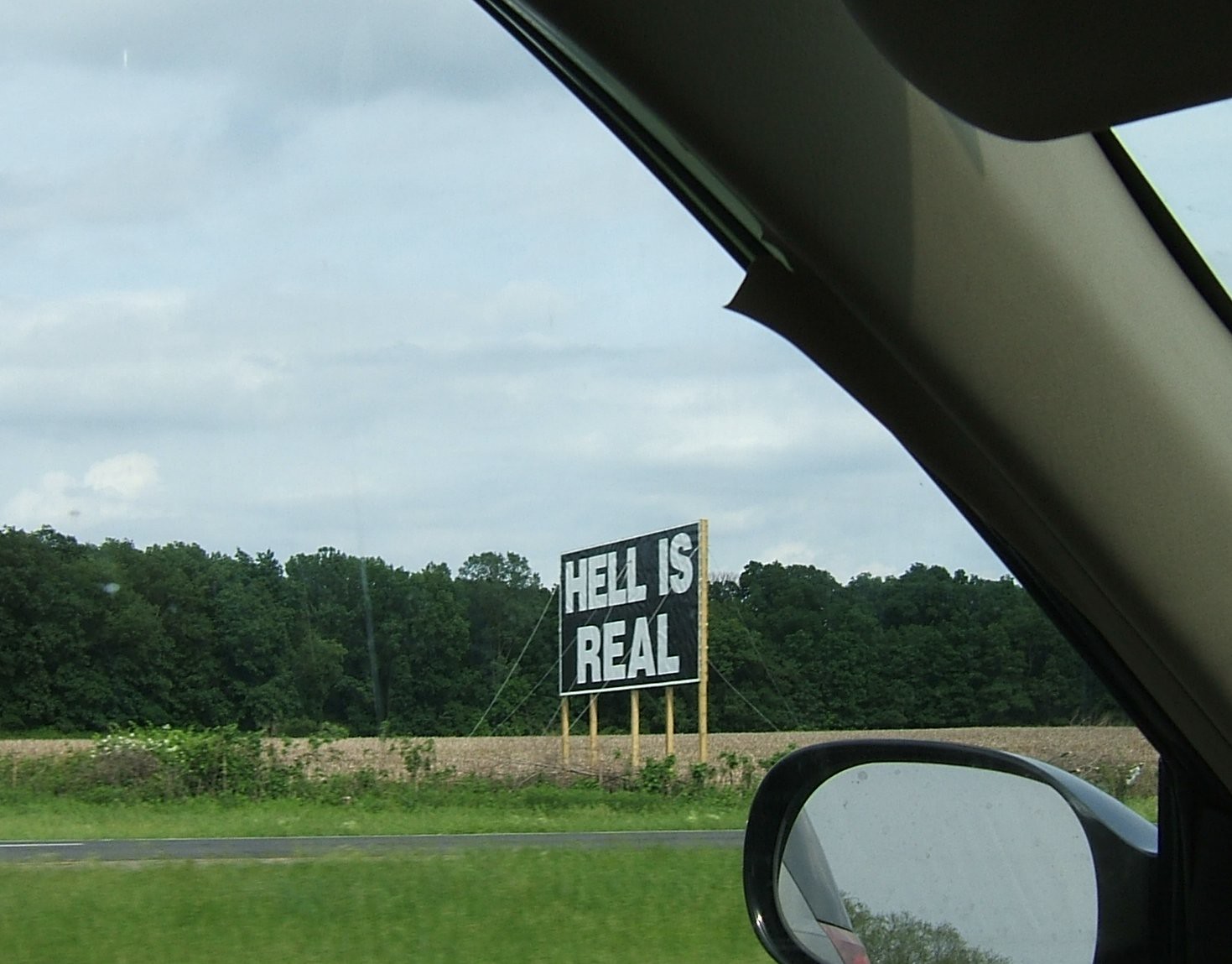A photograph taken from the driver's seat of a car reveals a detailed scene outside. The car, with a gray interior and a partially down window on the driver's side, has a black side mirror reflecting some trees and the edge of the vehicle with a red brake light visible. Through the window, a large billboard in the distance stands out in an open field, its black background adorned with stark white capital letters proclaiming, "HELL IS REAL." The dark green grass surrounding the sign transitions into lighter green and gradually gives way to a gray and gold field devoid of foliage. To the left, a dense line of tall, dark green trees forms a hedge-like barrier that towers over the sign, adding to the scene’s dramatic backdrop. The blue sky above is dotted with white and dark gray clouds, enhancing the natural contrast with the vivid greenery below.